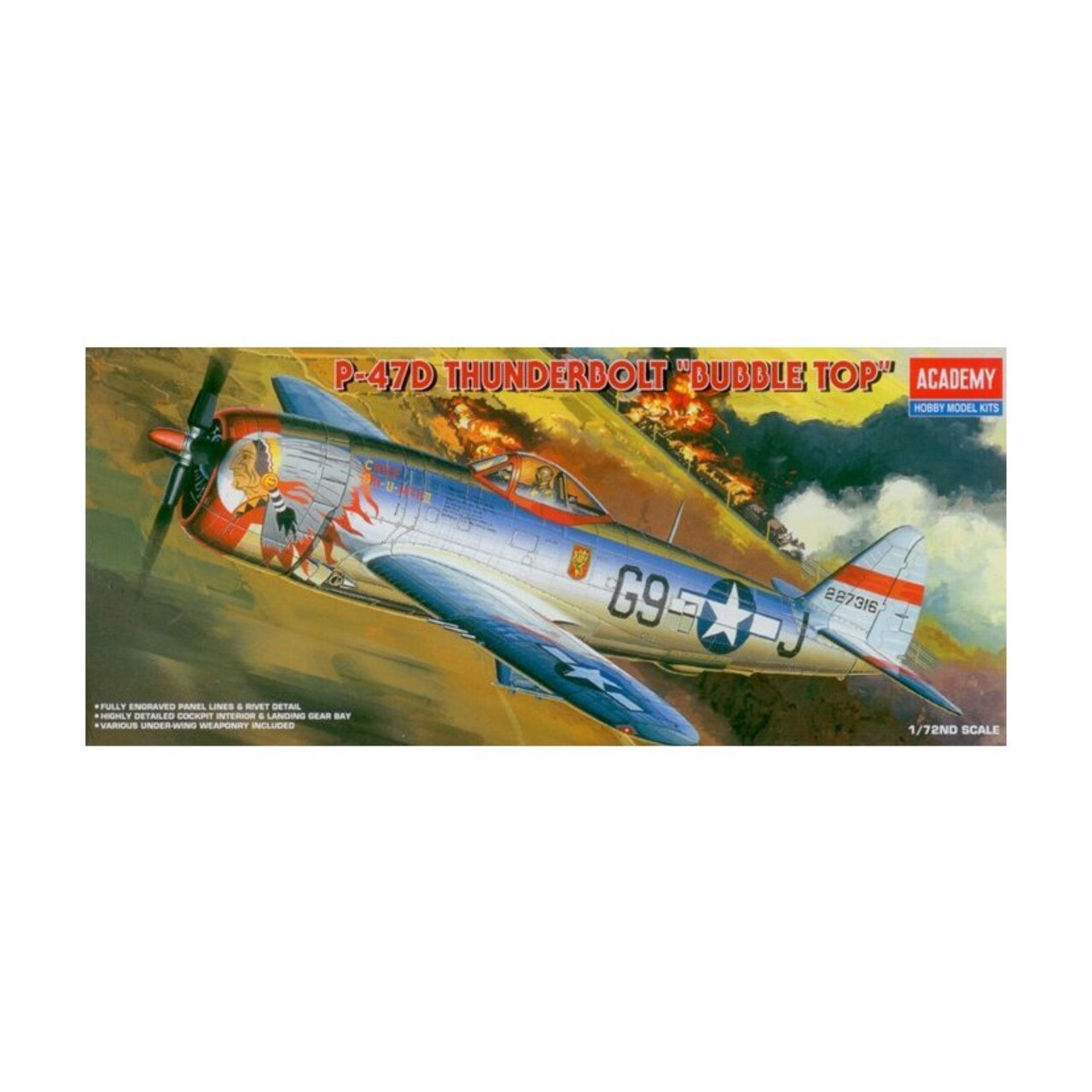The image is the cover of a 1/72nd scale model kit box for the P-47D Thunderbolt Bubble Top airplane. The box prominently features a hand-painted illustration of the aircraft flying over farmland with distant structures on fire. The silver-colored, propeller-driven fighter plane, designed in a World War II style, showcases several distinct markings: a Native American chief in a headdress just behind the propeller, the number G9 on the body, and white stars within blue circles on both the wings and fuselage. The cockpit is a bubble type, fitting a single pilot. The aircraft's tail displays the number 227316 along with a red stripe. The box is labeled in several places: “Academy” in white on a red rectangle at the top right, “Hobby Model Kits” in white on a blue rectangle below, and “P-47D Thunderbolt Bubble Top” in red with a white outline centered above the illustration.